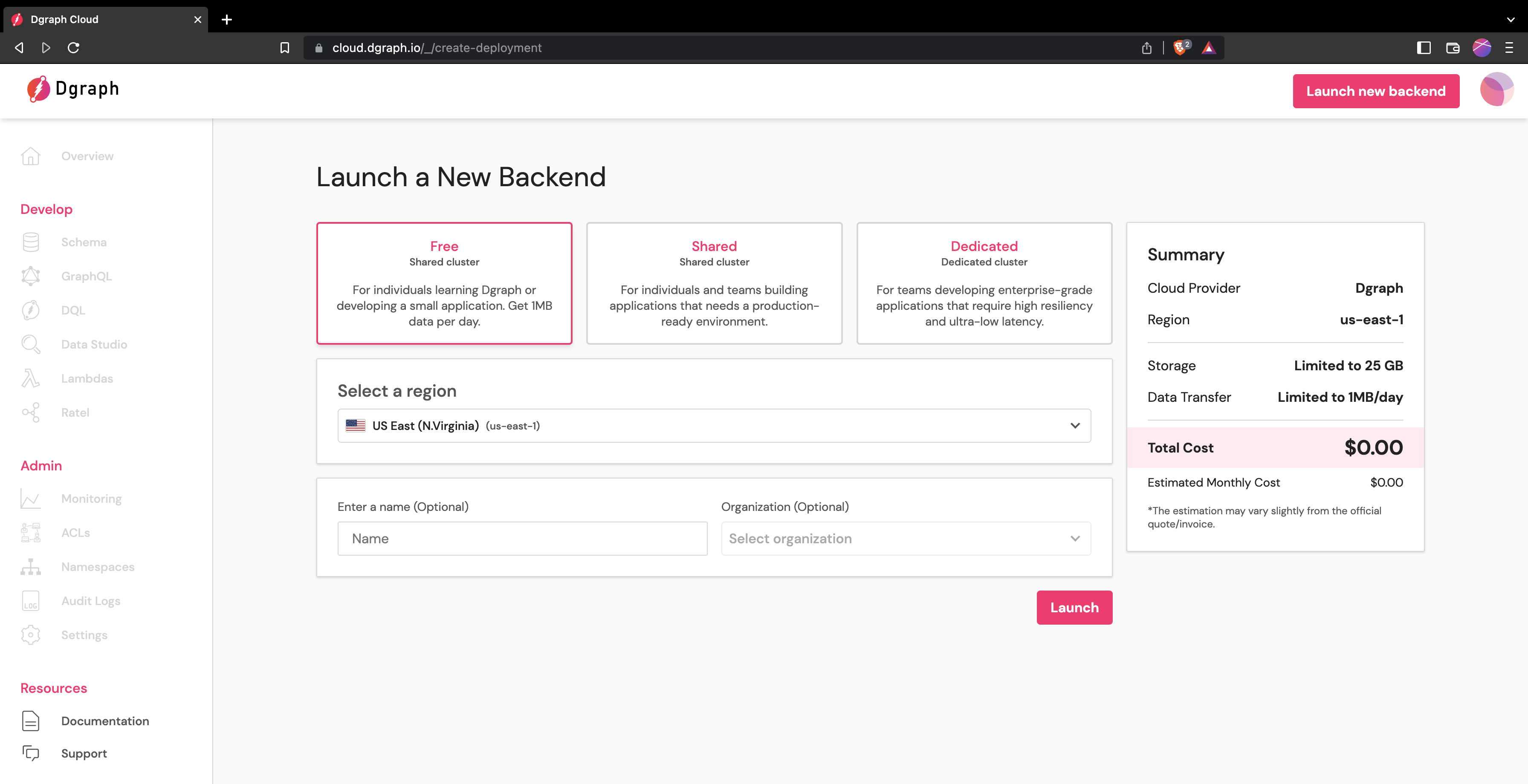In this detailed screenshot of the dGraph Cloud interface, the browser tab is open on the upper left-hand side, displaying the URL "cloud.dgraph.io/_/create/my/assigned/deployment." Dominating the right-hand side of the interface is a red button with white text that reads "Launch New Backend."

The main menu prominently features an option titled "Launch a New Backend." Below this, three distinct white boxes are visible, each offering different deployment options. The first box, outlined in a thin red border to indicate selection, is labeled for individuals learning dGraph or developing small applications. It offers a free shared cluster with an allotment of one megabyte of data per day. The middle box suggests a shared deployment, while the third box on the far right is dedicated. A launch button is also visible in the setup.